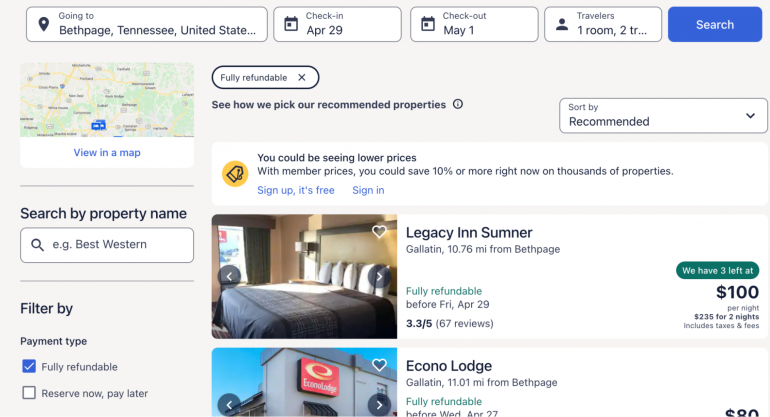The webpage describes properties, potentially hotels, in Bethpage, Tennessee, USA. At the top, there are several interactive boxes:

- The first box has a location icon and mentions "Bethpage, Tennessee, United States."
- Next, there are two calendar boxes for selecting "Check-in" (April 29) and "Check-out" (May 1) dates.
- There is a "Travelers" box featuring an icon of one person, indicating one room for two travelers.
- A blue "Search" button is provided for initiating the search process.

Below the search section, a map can be viewed by clicking on "View in a map." There is also a "Fully refundable" option next to a close button. Additionally, a note indicates, "See how we pick our recommended properties."

On the far right, there's a drop-down menu labeled "Sort by," with "Recommended" currently selected. A banner below this displays a message about potential savings: "You could be seeing lower prices." Accompanying this message is a yellow circle with a tag icon indicating membership benefits, stating that members can "save 10% or more right now on thousands of properties. Sign in, it’s free, sign up."

Below the banner, a property named "Legacy Inn Sumner Gallatin" is listed:

- Located 10.76 miles from Bethpage.
- Fully refundable before Friday, April 29.
- Rated 3.3 out of 5 stars based on 67 reviews.
- Only three rooms left at $100 per night or $235 for two nights, including taxes and fees.

Another property, "Country Lodge Gallatin," is mentioned:

- Located 11.1 miles from Bethpage.
- Fully refundable before Wednesday, April 27.
- Priced at $80 per night.

On the left, there’s a search box to find specific properties by name, with "Best Western" as an example. Nearby, filter options allow users to select "Fully refundable" or "Reserve now, pay later" payment types.